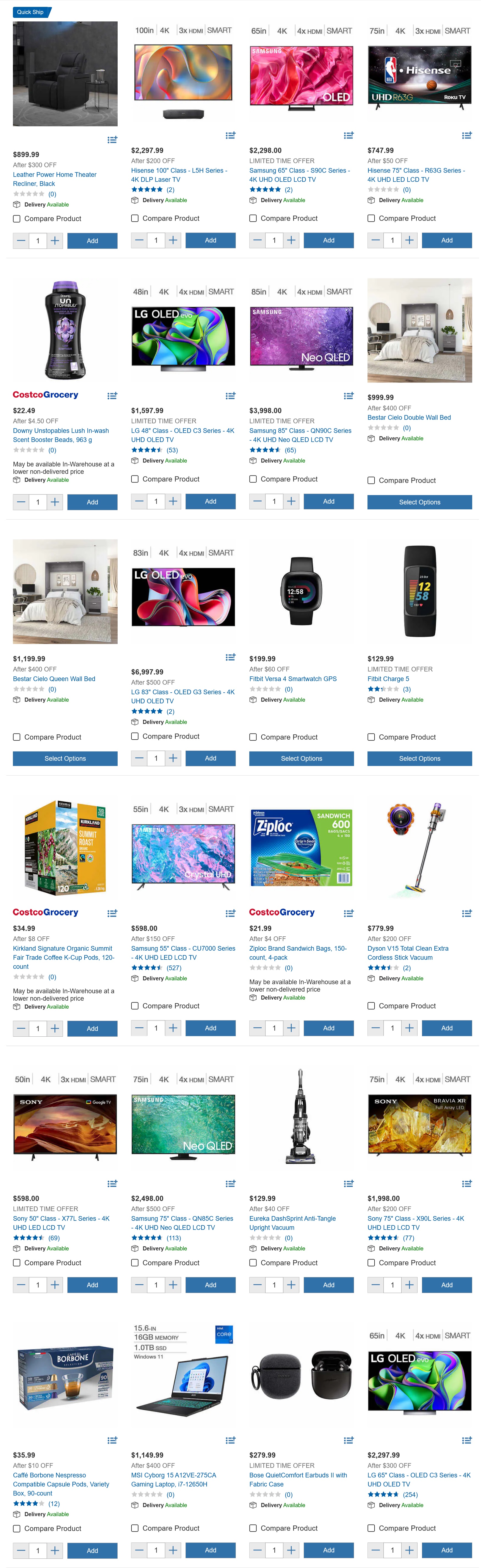A person is browsing an e-commerce website on their smartphone, which appears to be heavily focused on technology products. The interface lacks any visible header or browser chrome, making it challenging to identify the specific website. The screen displays a mock-up of a product grid that is too extensive to feasibly fit on a single phone screen, featuring a grid layout with four columns across and six rows down.

The visible products in the grid include a diverse range of items:
- **Row 1:** A chair and three televisions.
- **Row 2:** What appears to be shampoo next to a couple more TV screens and a bed.
- **Row 3:** Another bed, a TV screen, a smartwatch, and a phone.
- **Row 4:** Possibly software, another TV, Ziploc bags, and a Dyson vacuum cleaner.
- **Row 5:** Two more TVs, another Dyson vacuum cleaner, and yet another TV.
- **Row 6:** An unidentified product (possibly tea), laptops, earbuds, and a final TV.

Each product thumbnail is accompanied by its name, price, quantity selection options (adjustable with plus or minus buttons), and an "Add to Cart" button. Despite the detailed layout, the text is too small to read product details clearly.